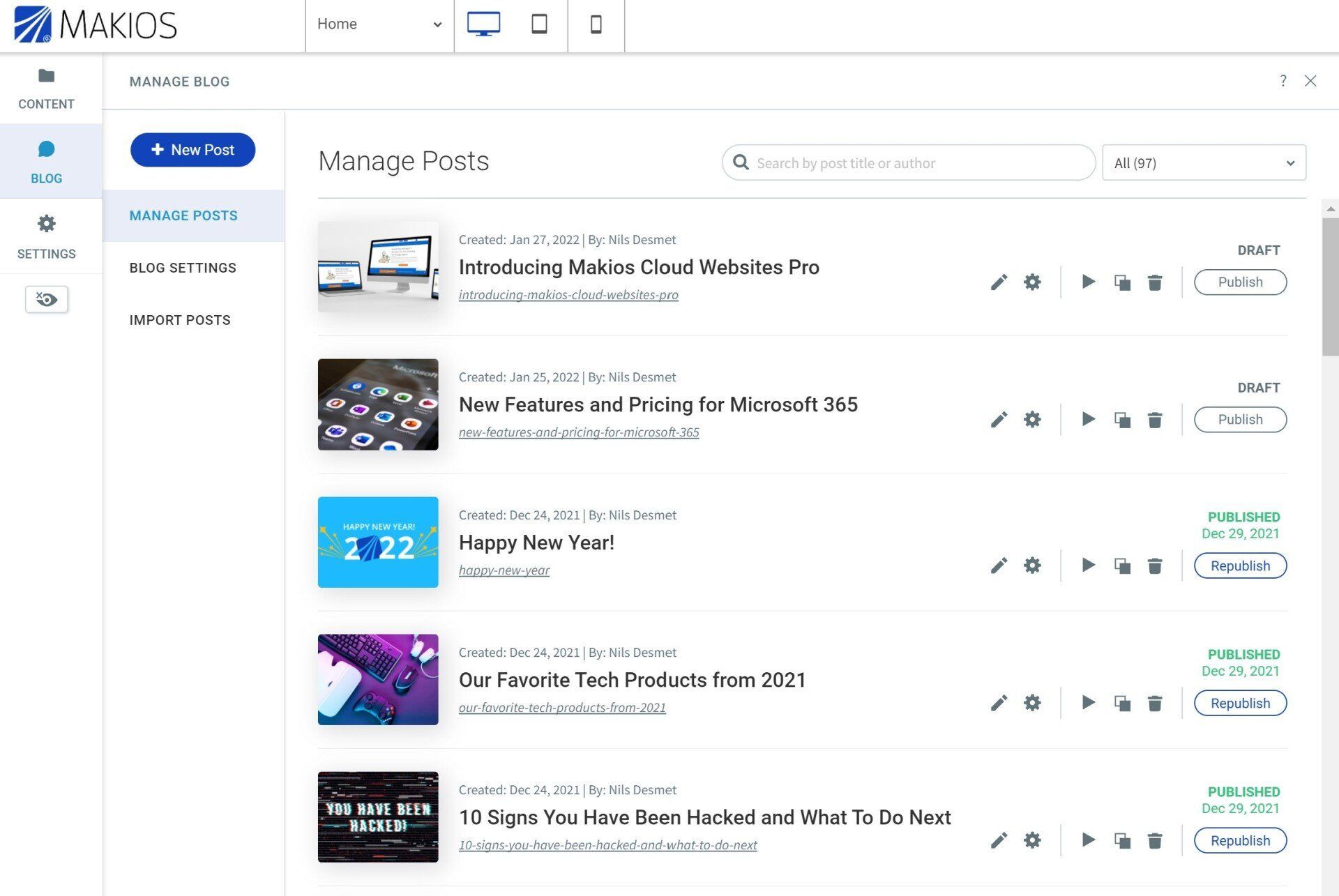This image is a screenshot of a blog management interface within a content management system, likely a part of a website's back end. The interface is organized into several sections, with the primary focus on managing blog posts. On the left side of the screen, a vertical navigation menu offers options such as Content, Blog, Settings, and Import Posts. Within the Blog section, it is expanded to reveal 'Manage Blog' and 'Manage Posts,' with the latter currently selected. A prominent 'Create a New Post' button is also visible.

The main display area shows a list of blog posts, each accompanied by details like the creation date, author, and status (e.g., published or draft). The posts feature titles such as 'Introducing MakeOS,' 'Cloud Websites Pro,' 'New Features and Pricing for Microsoft 65,' 'Happy New Year,' and 'Our Favorite Tech Products from 2021.' The interface is designed to provide an efficient way to oversee and organize blog content.